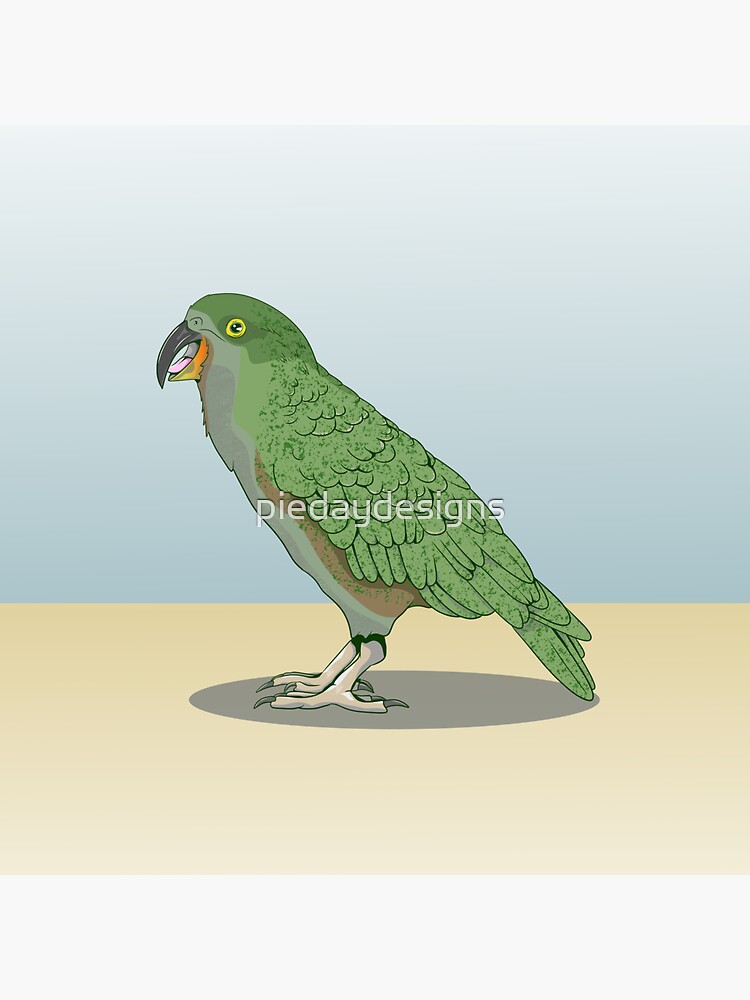A vibrant cartoon illustration depicts a green parakeet sitting atop a beige bar, possibly resembling a table surface. The parakeet's green feathers cover most of its body, with a darker green top of the head and darker green speckles on the wing feathers. The bird's black beak contrasts with a distinctive orange-colored lower beak and a visible pink tongue. Its eye is striking with a yellow hue surrounding a black iris. The bird's neck and belly are shaded grey, while a hint of brown is visible beneath the green wing. The background transitions from a soft pink at the very bottom to a gradient of light blue to white towards the top, providing a soothing backdrop that complements the bird's colors. An oval grey shadow directly beneath the parakeet adds a sense of depth to the image. A watermark reading "Pi Day Designs" in semi-transparent white text is centered within the picture, subtly marking the artwork.